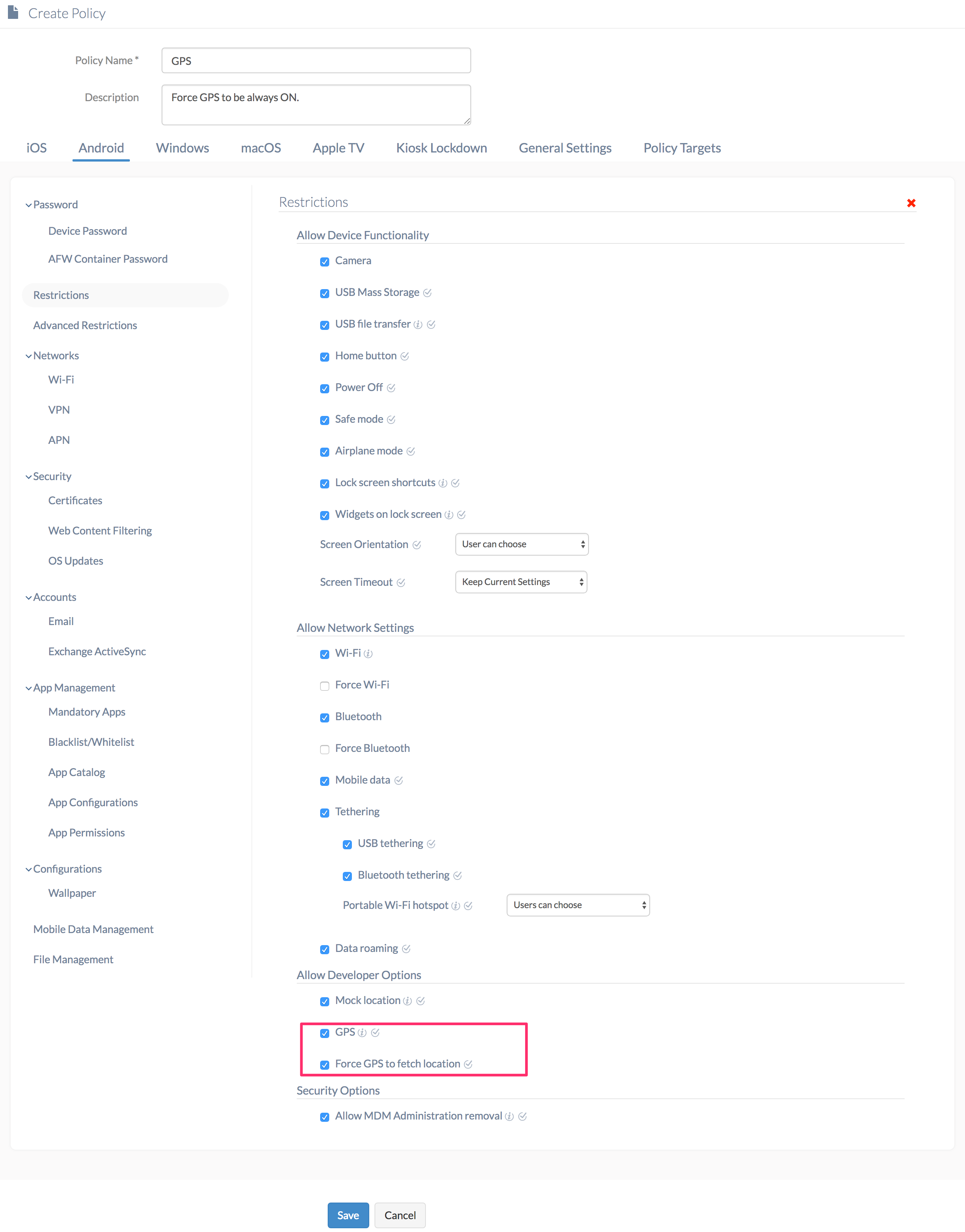This image captures a detailed settings screen of a device policy management interface. The policy name is "GPS," and it includes a description to force GPS to always be on. The interface is divided into several tabs: Android, iOS, Windows, MacOS, Apple TV, kiosk lockdown, general settings, and policy targets. 

Under the "Allow Device Functionality" section, the following settings are specified:
- Camera: Enabled
- USB Mass Storage: Enabled
- USB File Transfer: Enabled
- Home Button: Enabled
- Power Off Safe Mode: Enabled
- Airplane Mode: Enabled
- Lock Screen Shortcuts: Enabled
- Widgets on Lock Screen: Enabled
- Screen Orientation: User can choose
- Screen Timeout: Keep current settings

In the "Allow Network Settings" section:
- Wi-Fi: Enabled
- Force Wi-Fi: Disabled
- Bluetooth: Enabled
- Force Bluetooth: Disabled
- Mobile Data: Enabled
- Tethering: Enabled
- USB Tethering: Enabled
- Bluetooth Tethering: Enabled
- Portable Wi-Fi Hotspot: User can choose
- Data Roaming: Enabled
- Mock Location: Enabled